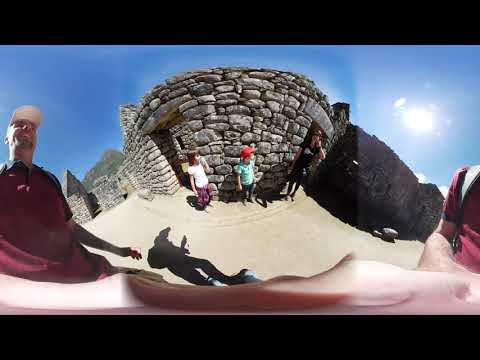This is a small horizontal rectangular image taken outdoors under a bright blue sky. The photograph is highly distorted, likely due to a fisheye lens or some similar effect, creating a bubble-like, rounded appearance. The image has thick dark boundaries at the top and bottom, focusing on a stone structure in the center. There are three people standing in front of this structure, which appears to be a stone wall. 

On the left side, a person is visible wearing a red shirt and a baseball cap, their body is warped by the lens, extending from the left edge to the right edge of the image. Their arm seems distorted at the lower portion of the photo, with their shadow being more accurate on the ground. In the center, a person in a green shirt and red cap stands, while on the right side, a person in dark clothing is partly visible, with only their arm clearly discernable. The person on the left may be taking the selfie, causing the unnatural wraparound effect. In the right corner, there is a bright hotspot from the sun, adding to the high-contrast nature of the image. The scene, overall, appears out of focus and skewed, with the blue sky accentuating the daytime outdoor setting.